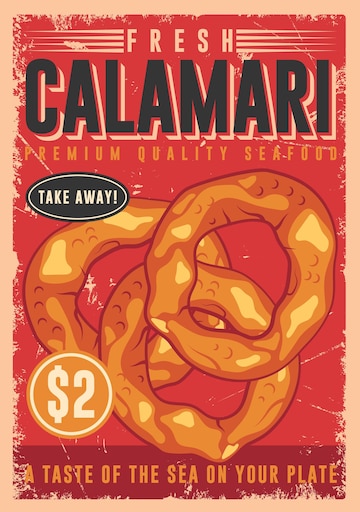The image is a vibrant yet worn and distressed poster primarily in red with a light tan or beige background. The top of the poster features the text "Fresh Calamari" in tan and black font, respectively, followed by "Premium Quality Seafood" in orange. The central graphic showcases a cartoonish, cel-shaded illustration of three rings of calamari. An oval positioned at the top left of the calamari rings contains the word "Takeaway" in black, while a yellow circle beneath on the bottom left indicates the price of "$2." At the bottom of the poster, a maroon bar with orange text reads, "A Taste of the Sea on Your Plate." The edges of the poster are visibly distressed, showing scratches and cracks, giving a worn, vintage feel to the artwork.